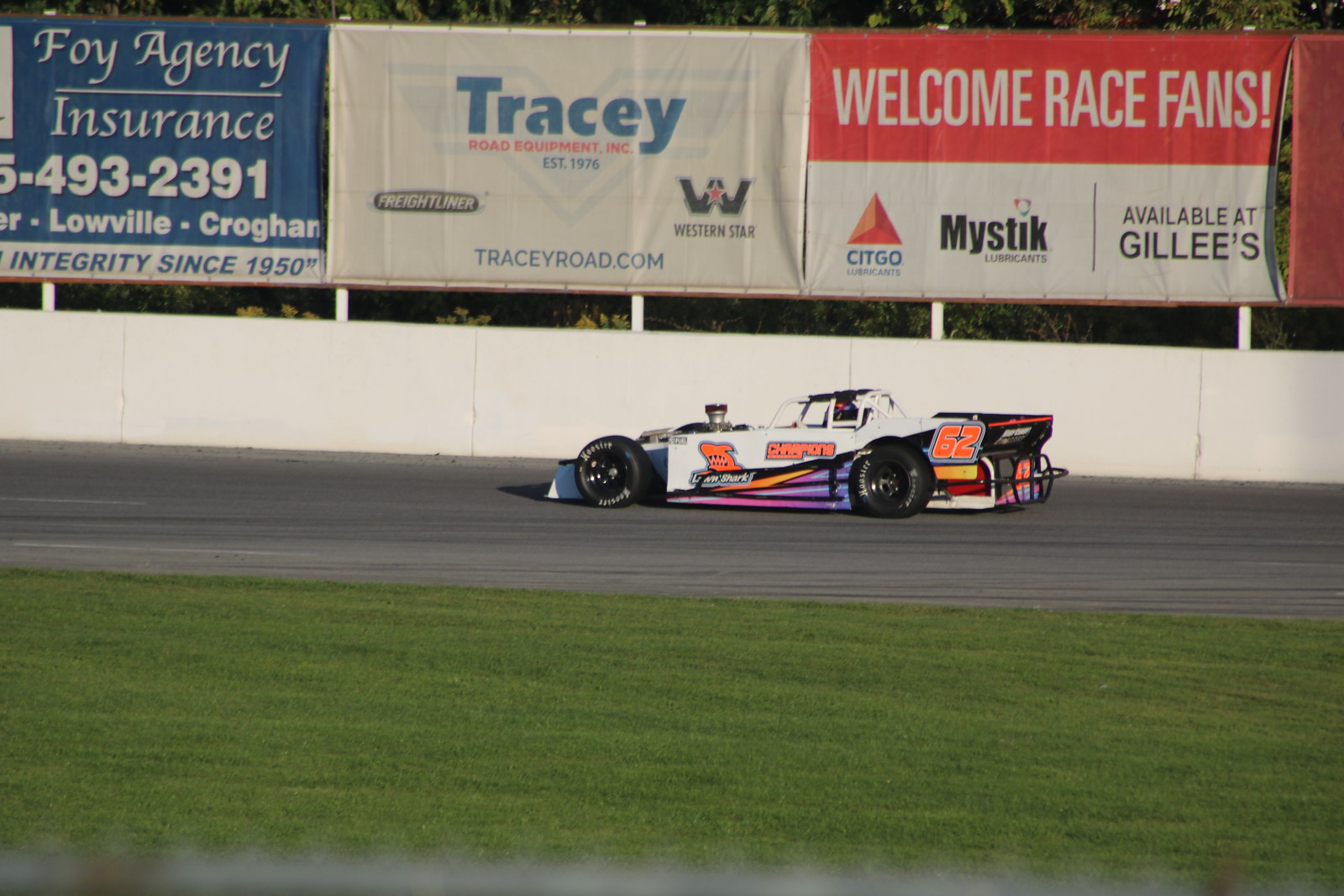The image captures a moment at a racetrack featuring an amateur Indy-style race car with a distinctive number 62 boldly displayed in orange on the back left side. The horizontal, rectangular photo shows the car in motion on a gray asphalt track with a green grassy infield in the foreground. The small race car, characterized by exposed black wheels, a sloping front end, visible roll cage, and a cab for the driver, is predominantly white with blue and orange trimmings, and a colorful graphic stripe down the side.

Adjacent to the path of the car is a white wall, nearly double the car’s height. Beyond this barrier, a series of large billboards loom overhead. On the left, a blue sign reads "FOIA Agency Insurance" along with a phone number. The center billboard features the word "Tracy" in blue on a white background, likely referring to Tracy Road Equipment Incorporated. The rightmost sign welcomes race fans with "Welcome Race Fans" emblazoned in red and white, alongside smaller logos for brands like Citgo and Mystic, indicating sponsorship and venue advertisement.